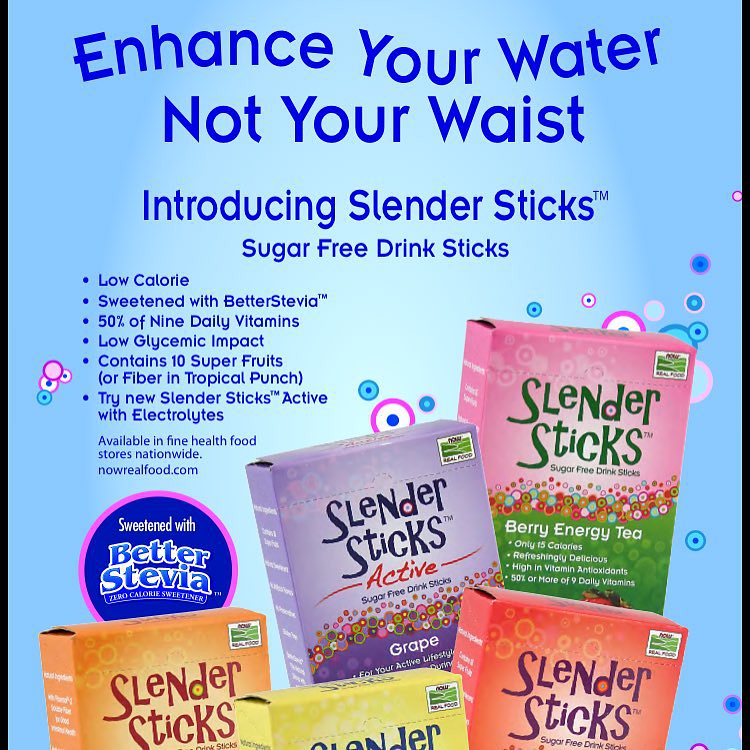The image is a digital brochure for Slender Stix™, showcasing a vibrant advertisement against a baby blue background with floating circles in various colors. Dominated by the tagline "Enhance your water, not your waste," the ad introduces these sugar-free drink sticks, highlighting their health benefits in bulleted points: low-calorie, sweetened with Better Stevia™, 50% of nine daily vitamins, low glycemic impact, and containing 10 super fruits or fiber in the Tropical Punch flavor. A call to action encourages viewers to try the Slender Stix™ Active with electrolytes, available at fine health food stores nationwide or nowrealfood.com.

The layout features five boxes of Slender Stix™ in different flavors and colors: "Active," "Berry Energy Tea," and visible ones in purple (Grape), pink and green, orange, yellow, and reddish-orange. Overlaying the boxes is a circle with a pink border that reads "Sweetened with Better Stevia™ Zero Calorie Sweetener." The colorful circles and box designs contribute to the playful yet informative aesthetic of the ad, designed to attract health-conscious consumers.